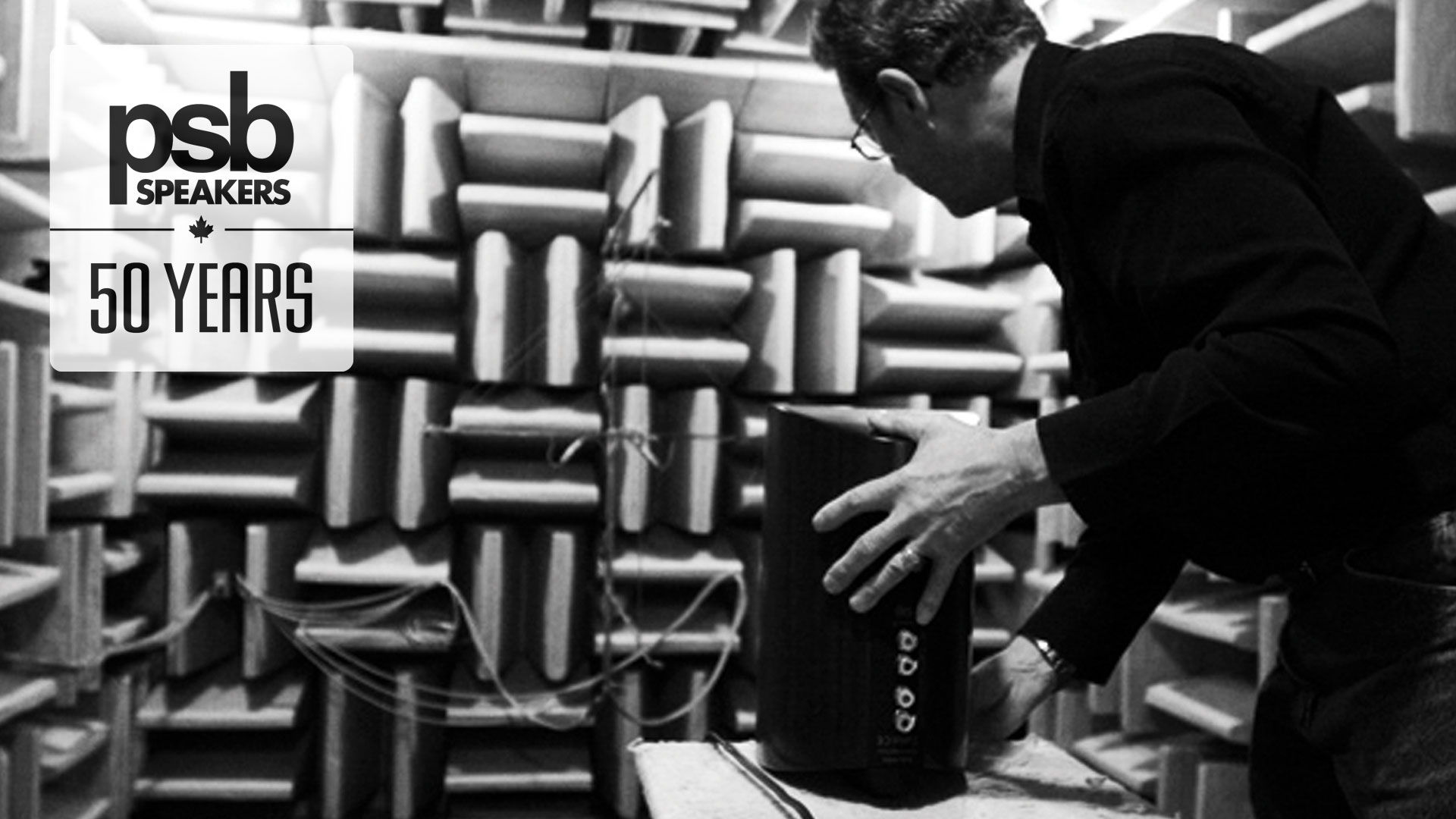The black-and-white photograph captures a man adjusting a black speaker. He is positioned to the right side of the image, wearing a long-sleeved black shirt, blue jeans, and glasses. His short hair frames a face that is looking away from us, revealing only a side and partial rear view. His hands are positioned around the speaker, one at the back and the other at the front, seeming to adjust its placement or connections. The speaker, facing away from us, shows various ports, including standard yellow-white RCA plugs.

The man is in a room designed with thin, rectangular acoustic panels protruding from the walls, likely to optimize sound quality and prevent noise escape. Cords and wires are visibly running in front of him, adding to the technical ambiance of the setting. In the upper left corner, a semi-transparent graphic box with rounded edges displays black text reading "PSB Speakers, 50 years," accompanied by a small Canadian maple leaf logo, indicating the company's Canadian heritage. The overall scene, possibly part of an advertisement, showcases the speaker and alludes to the brand's long-standing history and expertise in audio equipment.